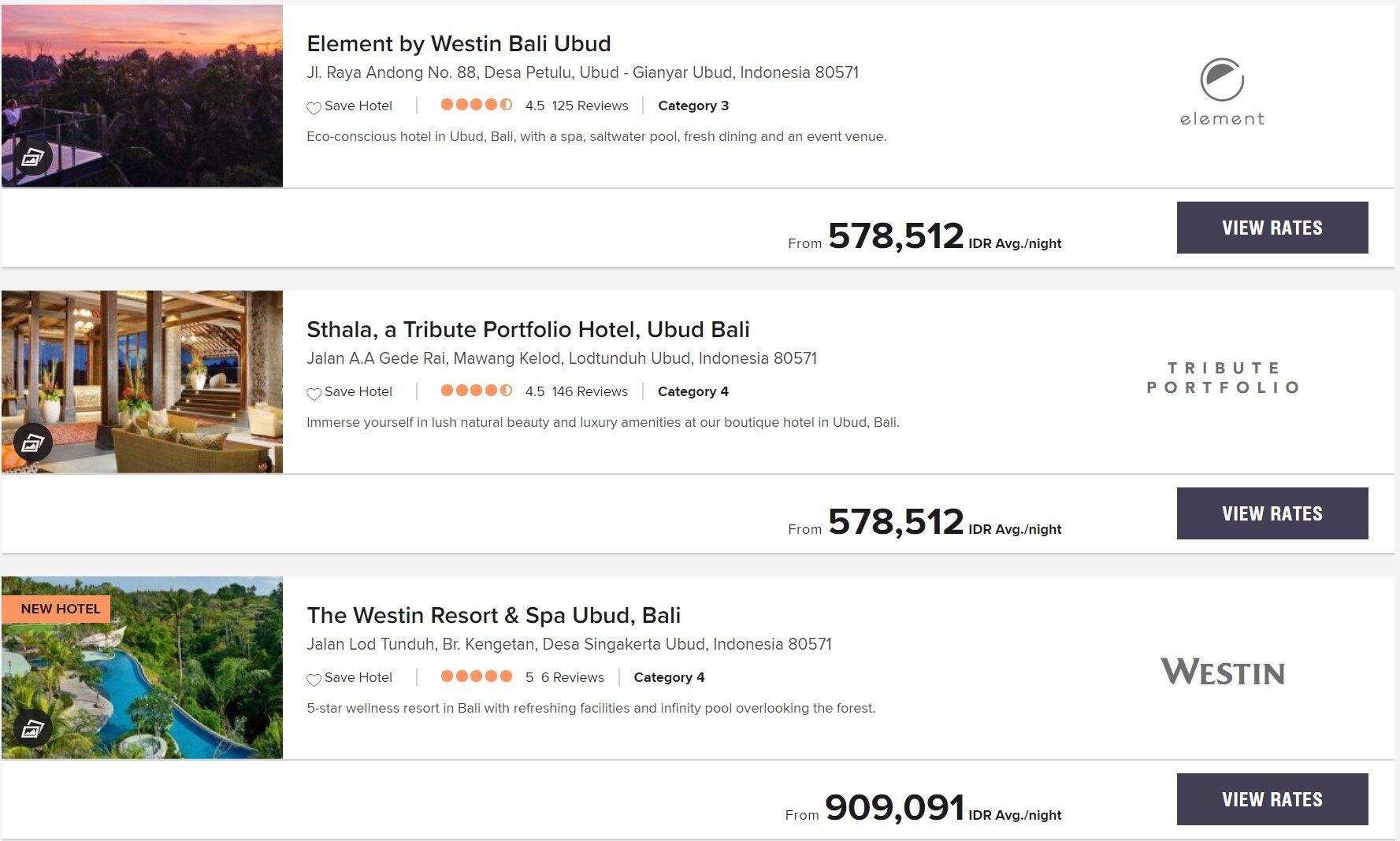This image is a screenshot from a web page dedicated to selecting vacation destinations, showcasing a clean and minimalist design with a predominantly white background. The page features three distinct options, each representing a different hotel or spa, appealing to potential vacationers.

On the left side of the screen, there are photographs of each location, providing a visual preview of the destinations. To the right of these images, detailed descriptions of the locations are provided. These descriptions are accompanied by rating indicators, which are depicted as circles; the first two options have ratings of 4.5 circles, while the third option boasts a full 5-circle rating.

Additionally, next to each description on the far right, there is a dark blue button labeled "View Rates." This button invites users to click and access more detailed pricing information for each respective destination.

Specifically, the top option is identified as "Element by Westin Valley Ubud," underlining its potential as an appealing destination for travelers. Overall, the page effectively organizes the information, making it easy for users to compare the various vacation locations and their respective ratings.